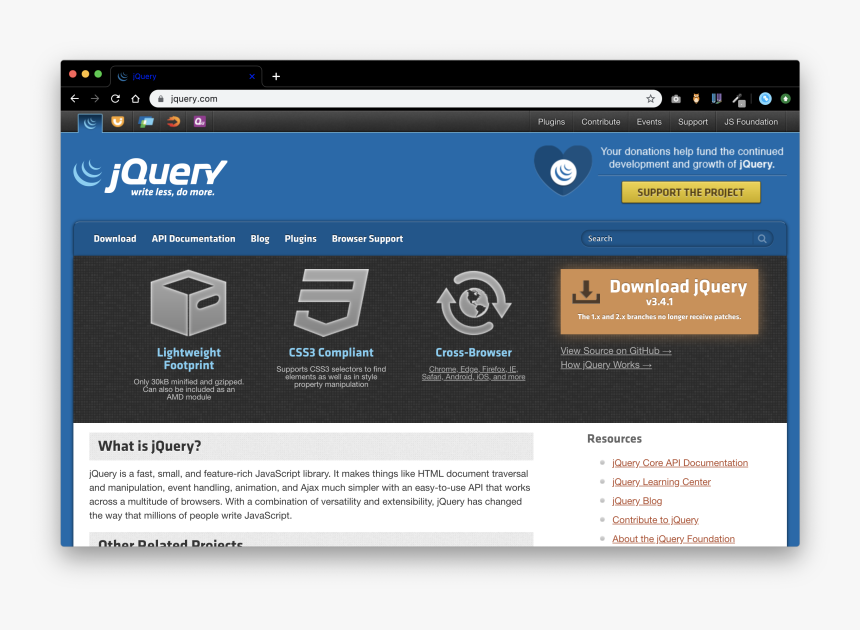A detailed web page caption:
 
The image displays a web browser open to the homepage of jQuery's website, accessed via entering "jquery.com" in the search bar. The jQuery logo is prominently placed in the upper left corner, accompanied by the tagline "Write Less, Do More."

To the upper right, there is a notice urging users to donate to support jQuery’s development, accompanied by a yellow rectangular button labeled "Support the Project." Above this section, the navigation menu includes links labeled "Plugins," "Contribute," "Event Support," and "JS Foundation."

Central to the page, several headings in white text stand out, including "Download," "API Documentation," "Blog," "Plugins," and "Browser Support." Beneath these headings, a series of icons and brief descriptions provide additional information. The descriptions read, "Lightweight Footprint" under the first icon, "CSS3 Compliant" under the second icon, and "Cross Browser" below two small arrows.

A notable feature on the right side of the page is a yellowish-orange rectangle with text that prompts users to "Download JQuery v3.4.1."

At the bottom of the page, against a clean white background, there is a heading that says "What is jQuery?" followed by a detailed paragraph explaining the nature and purpose of jQuery.